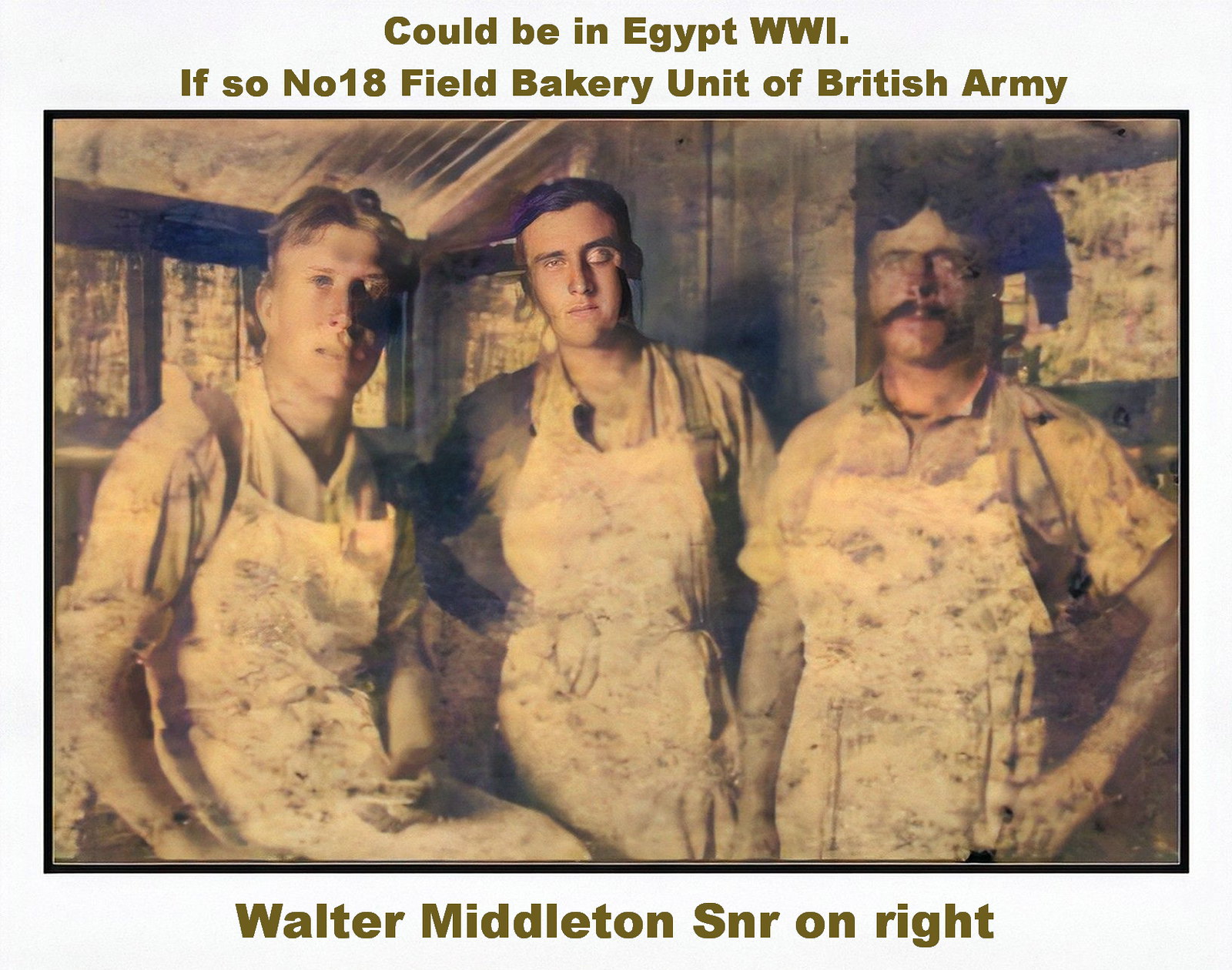This vintage photograph features three men, possibly bakers from the British Army's 18th Field Bakery Unit during World War I, standing in front of a rustic wooden structure that resembles a hut or kitchen. The image, which has a light blue border with the text "Could be in Egypt, World War I, if so, Number 18 Field Bakery Unit of British Army" at the top, and "Walter Middleton SNR on right" at the bottom, is sepia-toned with some colorization, especially noticeable in the men's skin tones. Two of the men are clean-shaven, while the third sports black hair and a matching mustache. All three are dressed in colored shirts beneath white aprons, with their hands by their sides, facing the camera from the waist up. The photograph, which appears worn and stained with visible imperfections, evokes a sense of fatigue and toil, hinting that they may have been in the midst of preparing or finishing up a meal.